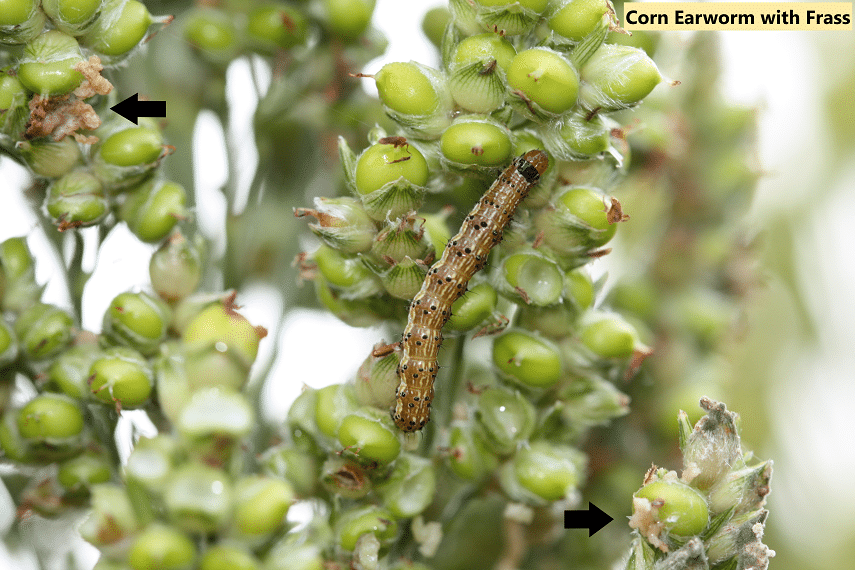In this detailed image, there is a close-up view of green grapes or berries clustered on a vine. Among the berries, a long, smooth, tannish-brown caterpillar, identified as a corn earworm, is prominently visible. The background appears to be out-of-focus foliage, matching the plants in the foreground, thus providing a greenish tint throughout the image. Labeling in the upper right-hand corner, enclosed within a yellow box with black text, confirms the presence of the "corn earworm with frass." Several black arrows are present in the image: one in the upper left points towards possible larvae, and another in the lower right corner directs attention to a smaller detail, possibly another larva. The entire scene encapsulates a garden or agricultural environment, focusing particularly on the infestation of the corn earworm.